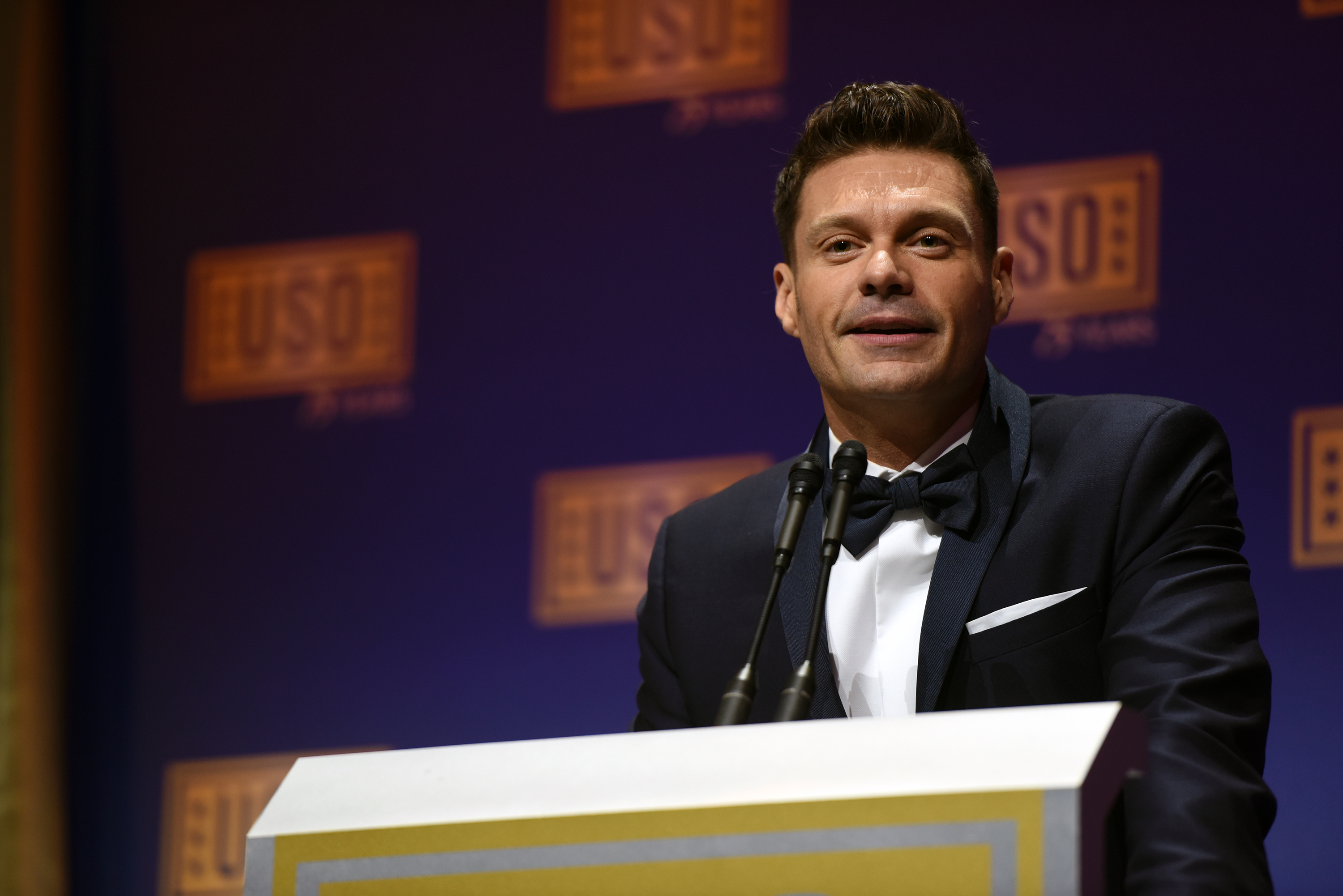This color photograph features the celebrity and presenter Ryan Seacrest, who is well-known for his roles as an emcee and host. He is captured from an audience perspective, standing confidently behind a metallic silver podium adorned with a yellow border, and equipped with two small microphones. Seacrest is dressed impeccably in a black tuxedo paired with a white dress shirt, a black bow tie, and a neatly folded white pocket handkerchief. He is smiling and looking downwards, presumably engaging with the audience while delivering a speech. The backdrop behind him is a dark blue banner with gold lettering that prominently displays the logo "USO," suggesting his involvement in a USO event. His short hair is neatly styled, adding to his polished appearance for the formal occasion.